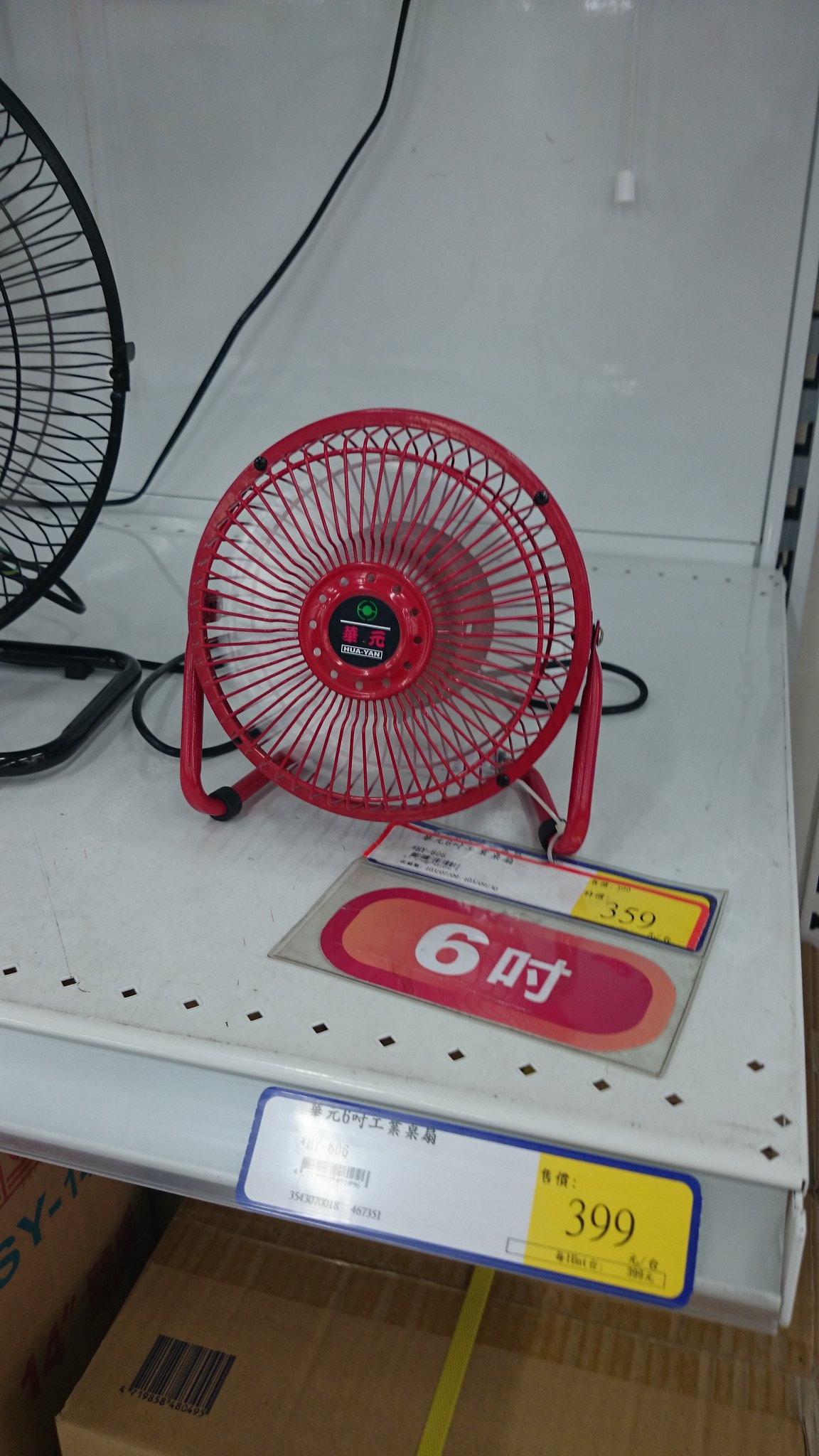The image showcases a shop shelf featuring two fans available for purchase. On the left side, there's a large black fan plugged in with a long black cord extending from behind. It has detailed Chinese lettering indicating a size of 6 inches and a price of 3.59 yuan. Adjacent to the black fan, on the right, resides a small red fan, standing no taller than 3-4 inches. The red fan's structure allows visibility of its internal blades, and it rests on a steel-frame stand. Below the fans, a white shelf with little holes along its edge supports another sign in yellow with black writing, displaying a price of 3.99 yuan. Additionally, there are sealed cardboard boxes beneath the shelf, which likely contain the fans for sale.